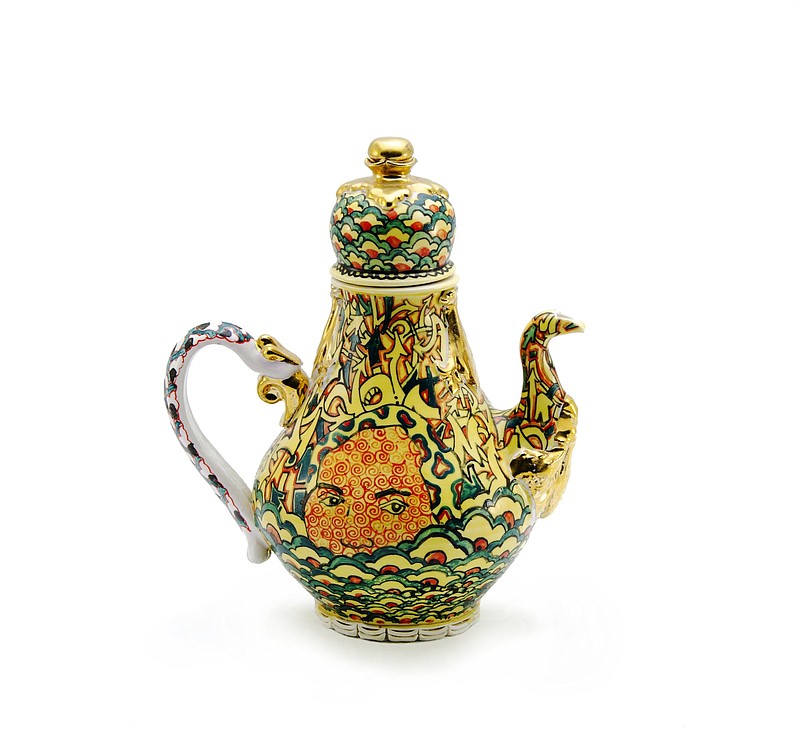This photograph showcases an ornate porcelain teapot set against a white background on a white table. The teapot is a vibrant canvas teeming with an elaborate and multicolored design featuring yellows, greens, blues, reds, and oranges. The top cap of the teapot has a golden handle with intricate details extending down over the porcelain. Both the top and bottom of the teapot display consistent patterns of green borders, a yellow band, and a red center, mirroring each other. A prominent face is painted in the middle of the teapot, composed of forehead, eyebrows, eyes, nose, and cheeks, partially obscured by swirling red patterns reminiscent of graffiti. This face merges seamlessly into flower motifs with green-blue petals and red centers that adorn various parts of the teapot.

The spout of the teapot is distinctively shaped to resemble a bird, complete with golden embellishments and similar patterning to the rest of the pot. The handle is primarily white with green decorations and attaches to the back of the teapot with golden details, curving elegantly downwards. Overall, the teapot's surface is densely ornamented with no space left untouched, presenting a royal and whimsical appearance. Shadows beneath the teapot suggest it is lit from above, enhancing its majestic and busy aesthetic.